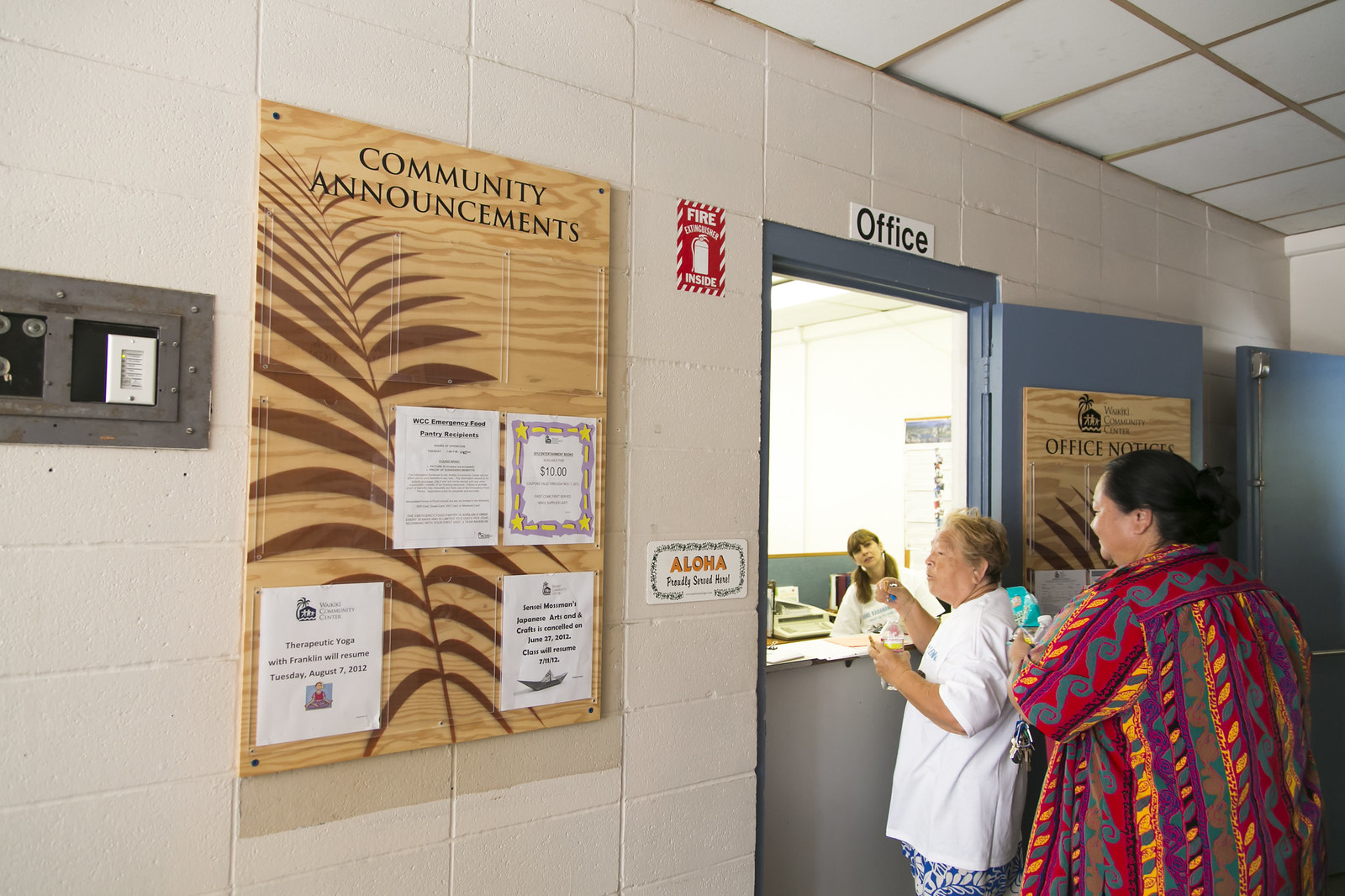The image depicts two women visiting an office. The scene shows them standing at a counter to conduct some business, while a lady is behind the counter on the opposite side. Above the window at the counter, a sign reads "Office" and is affixed to a tan-colored cement wall. To the left of the image, a wall-mounted community announcement board made of wood features a fern design and holds several white pieces of paper, though the text on them is unreadable. Directly to the right of this is a sign indicating a fire extinguisher, and below it is an "Aloha" sign positioned by the door. Hanging from the door is another wooden sign with a leaf that reads “Office Notices.” The woman closest to the counter wears a white shirt and blue pants and seems to be holding a cup, with her brown hair visible. Behind her stands a second woman in a vibrant, colorful dress in hues of blue, yellow, orange, green, and black, with black hair.